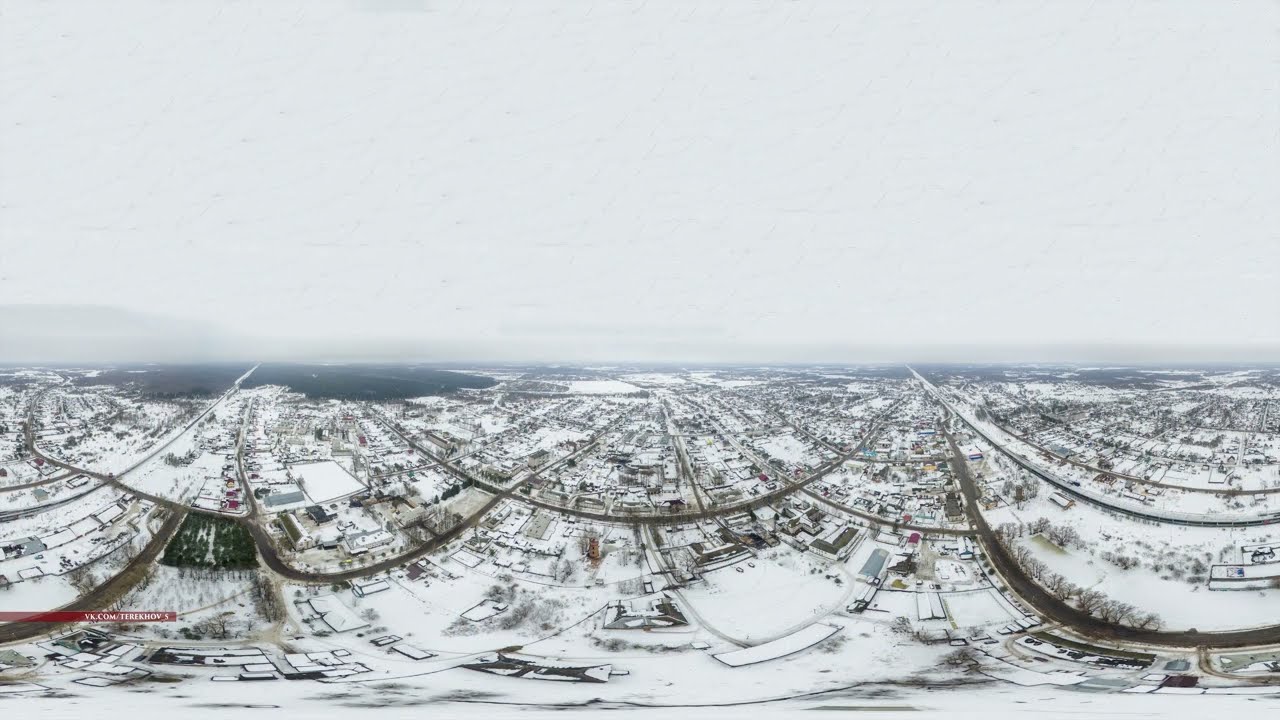This image presents a digitally altered, panoramic aerial view of a snow-covered cityscape, characterized by a stretched and warped perspective. The scene is encased in a horizontal, rectangular frame, dominated by a dark blue sky with a prominent, thin white stripe resembling a cloud running across the center, giving the skyline a glowing effect. Below this horizon, the city sprawls towards the edges, showcasing a blend of cleared roads cutting through densely packed snow-covered buildings, from regular houses to apartment complexes. Interspersed among the structures are patches of dark green and barren trees, adding texture and contrast against the predominantly white landscape. The clear, grey roads intersect and converge towards the lower part of the image, highlighting the meticulous, almost surreal clarity of the winter scene. This image's unusual and exaggerated fisheye lens effect contributes to the sense of distortion, making the buildings appear bent and the overall vista almost dreamlike.